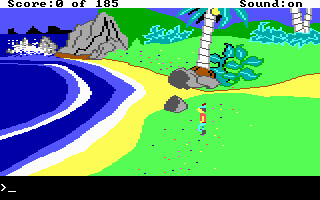The image appears to be a screenshot from a simplistic, likely 1980s-style video game, as indicated by its primitive, computer-generated graphics. At the top of the screen, text reads "Score: Zero out of 185" and "Sound is on." A blinking cursor at the bottom suggests the game is awaiting player input.

The scene depicts a beach setting rendered in a cartoon style. Blue water with white crests indicating waves dominates the left side, with a gray cliff in the background. In the center and extending to the bottom right is a sandy pathway, flanked by grass and greenery dotted with blue, yellow, and red hues. A small, cartoonish figure stands on this pathway, appearing to march toward the beach. A prominent palm tree, complete with fallen coconuts, marks the transition from grassy area to sand. Further back, beyond the tree, the terrain appears to lead to additional grassy areas and rocks, possibly containing small houses and a canoe near the water's edge. The sky is bright blue, and there are shadows cast behind the rocks, adding depth to the scene.